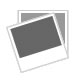The photograph features an antique songbook titled "Sing a Song of Sixpence," open on a table amidst several other books. The well-worn pages are yellowed with age and exhibit muted, almost faded colors. The left page displays the song's title along with musical notes and lyrics printed beneath in black, flowing from the left to the right page. Scattered illustrations complement the music, including black crows, a king in a red robe and yellow crown preparing to carve a pie, and a queen in a green robe partaking in a feast. On the right page, the same king is depicted in pajamas, counting a heap of gold with a green treasure chest nearby. Notably, a frightened blonde woman in a white and blue dress appears in the bottom right corner, being harassed by a crow. The book, set atop a pile of others, stands out as the primary focus in a setting that reveals additional music books and some kind of hosing in the background.